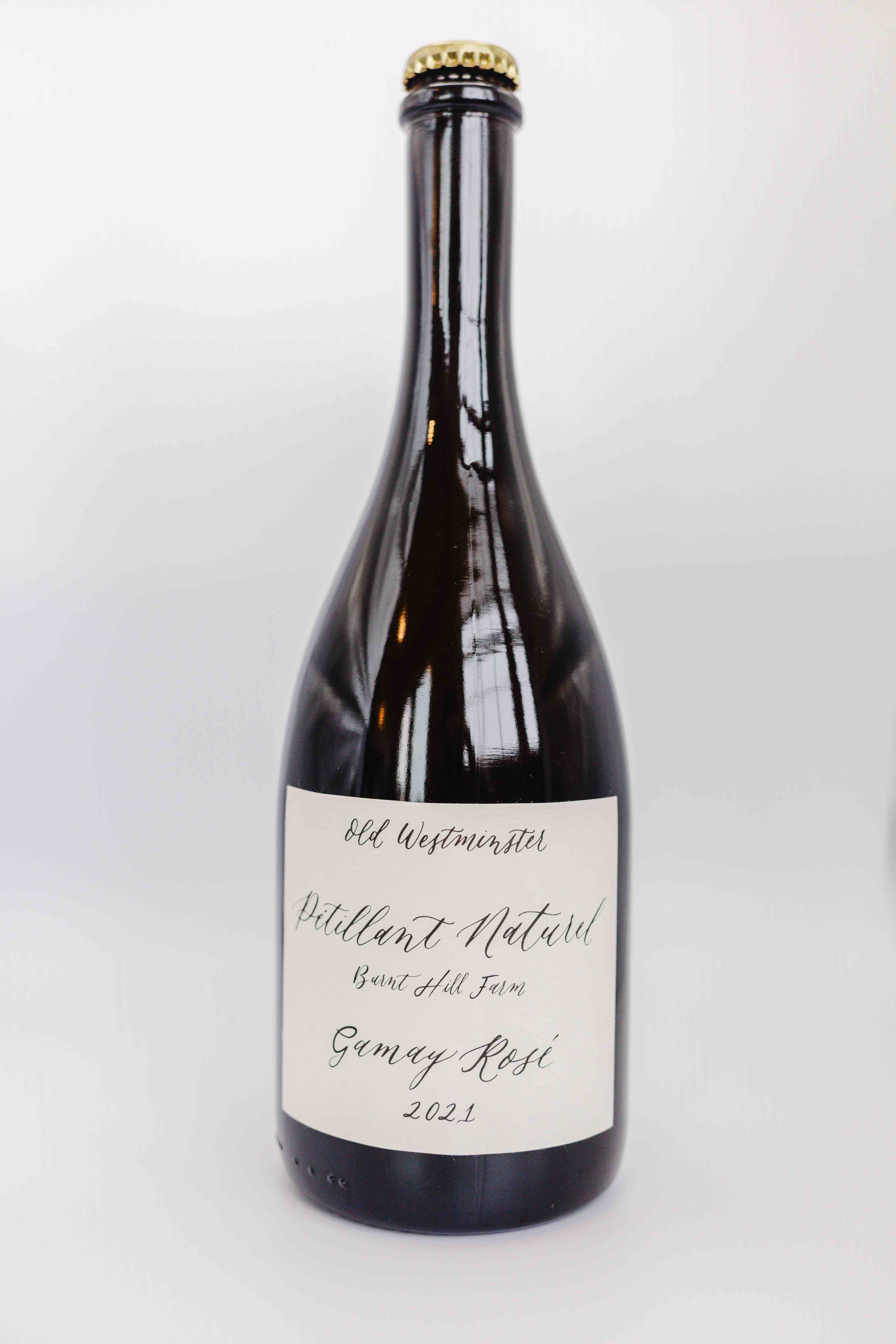The image features a dark-colored, possibly black, glass bottle, indicative of wine, with a long neck and a screw top, which appears to be metallic, likely gold. The bottle prominently displays a minimalist white label with elegant cursive writing that reads "Old Westminster." Beneath it, the label further details "Pétillant Naturel Burnt Hill Farm" and "Gamay-Rossi 2021," though the precise wording is slightly obscured. The bottle reflects a significant amount of light, revealing the faint outline of the photographer, specifically their legs and torso, in the glare. The backdrop is a plain whitish-gray, offering no distinct surface but highlighting the bottle's rich, dark glass and the stark contrast of its white label with black text.